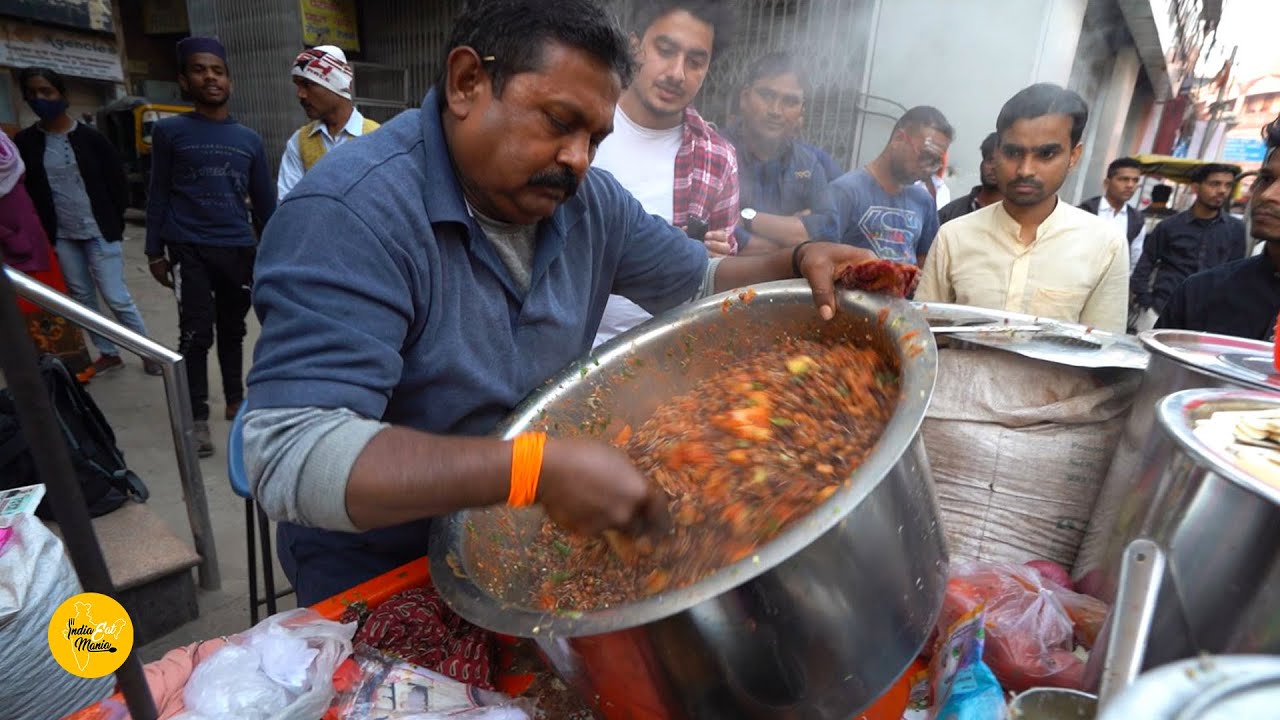An elderly gentleman, likely of Indian descent, is captured in this photo holding the largest metal pot I have ever seen. The scene appears to be outdoors in a modest setting, indicative of a less affluent area. The gentleman, dressed in traditional attire, seems to be preparing to serve a hearty stew, as visible inside the pot are substantial pieces of meat, green beans, and carrots. Surrounding him are about 15 to 20 young men, presumably waiting in line for their meal, suggesting a humanitarian effort to feed the homeless or those in need. Additional metal pots with lids are scattered around, hinting at a well-organized distribution. The image vividly portrays a moment of compassion and community support.